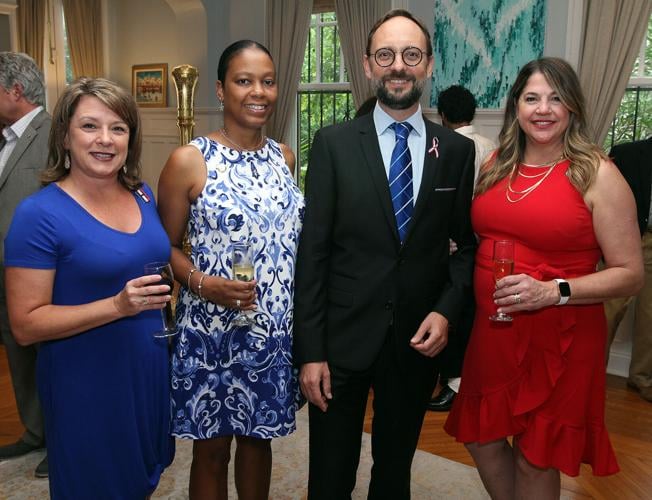In a warmly lit room with light beige walls, various art pieces adorn the surroundings. A gold pole is subtly visible in the background, alongside a window with decorative bars, framed by soft beige curtains. A notable painting on the wall features an intriguing combination of green, dark green, and white hues.

Four people occupy the foreground, all holding drinks and engaging in what appears to be a sophisticated gathering. The first is a lady dressed in a striking blue dress, holding her drink delicately. Next to her stands a black lady donning a stylish blue and white dress, also with a drink in hand. A gentleman in a sharp black suit with a complementary blue tie joins the group, alongside a lady in a vibrant red dress, drink in hand. 

In the background, a black gentleman in a crisp white jacket is captivated by the artwork on the wall. The scene is completed by another man at the far end, distinguished by his gray suit and matching gray hair. The entire ensemble captures an elegant moment of social interaction amidst a backdrop of cultured refinement.